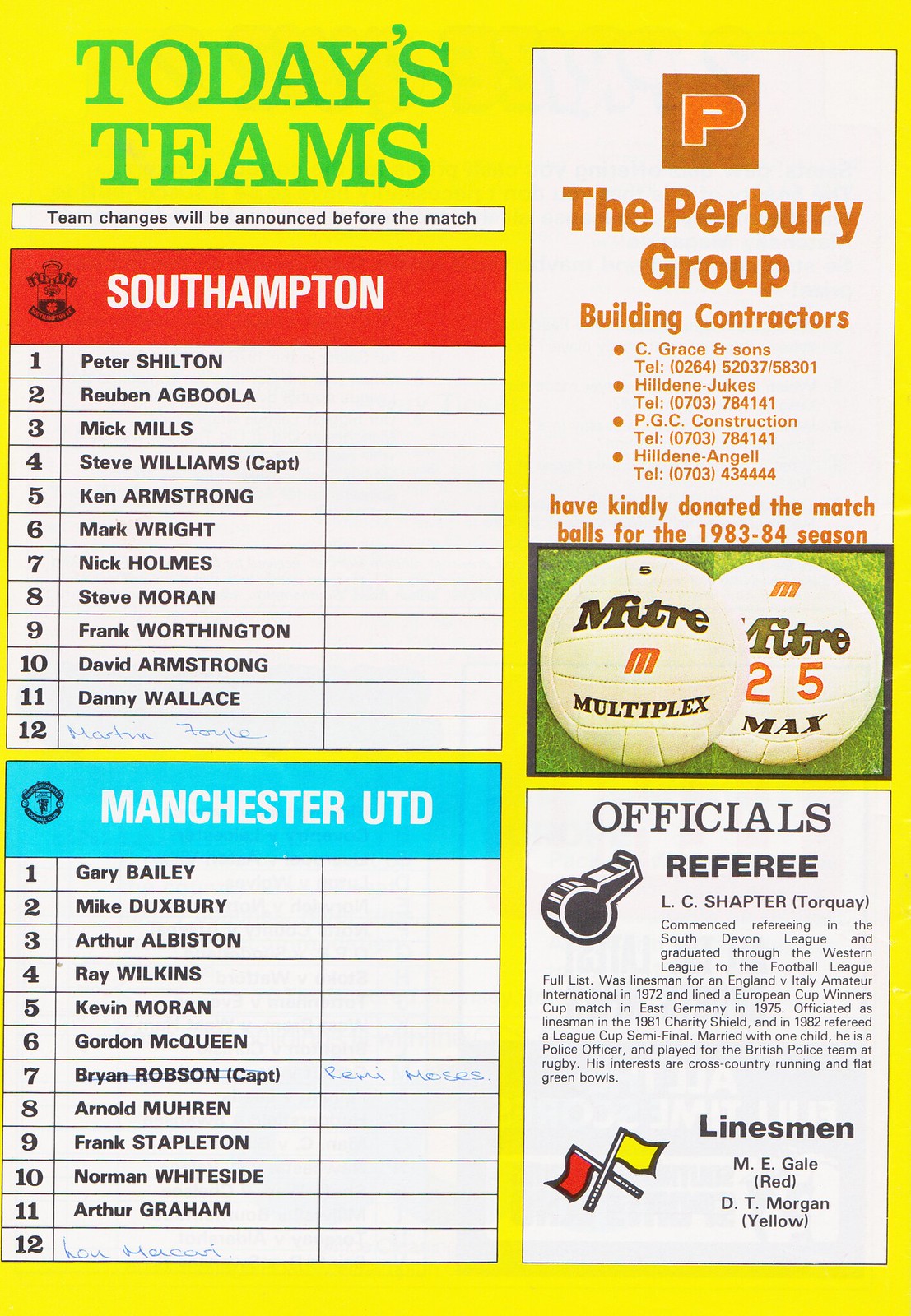The image displays a page from a British football (soccer) program. It features a yellow background with a prominent greenish header that reads "Today's Team" in the top left corner. Below the header, a note indicates that "team changes will be announced before the match." On the left side, the program highlights the two teams playing: Southampton, on a red background with white lettering, and Manchester United, on a light blue background with white lettering. Each team's player names appear beneath their respective headers, alongside blank boxes likely meant for spectators to jot down notes or indicate player attendance.

To the right, there is an advertisement for the Peaberry Group Builders Contractors in orangey-brown lettering. Another feature at the bottom of this section is an ad for Mitre soccer balls. Additionally, the page lists the officials, including the referee and linesmen, alongside a brief story about them.